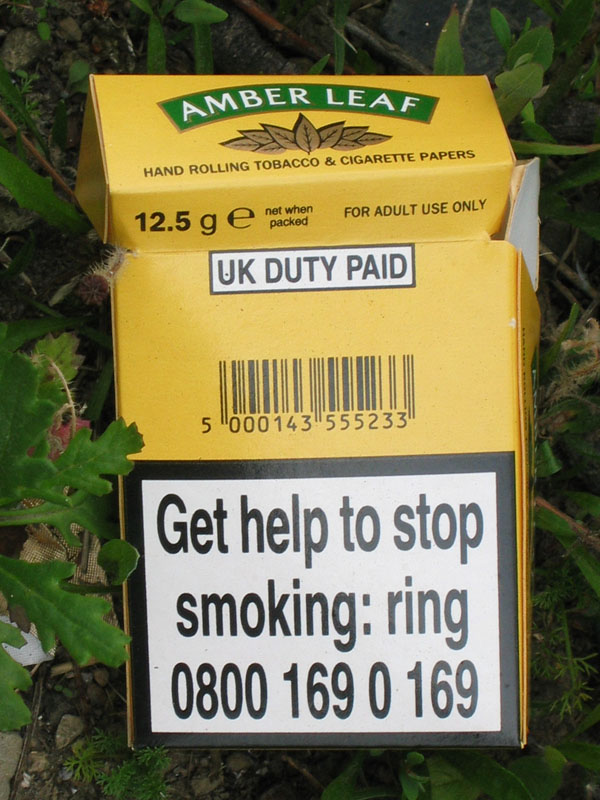This close-up image showcases a yellow package of Amber Leaf hand rolling tobacco prominently set against a lush, green backdrop of leafy plants and trees. The top of the package curves slightly and features the brand name "Amber Leaf" in green with white font. Beneath this, in black font, it reads "hand rolling tobacco and cigarette papers," followed by the specification "12.5 G E-net when packed" accompanied by the phrase "for adult use only." Further down, a white box outlined in black displays "UK duty paid" in capitalized black font, along with a UPC number "501435552333". At the bottom of the package, in a black-bordered white box, there is a message in bold black font: "get help to stop smoking ring 0800-169-0169."